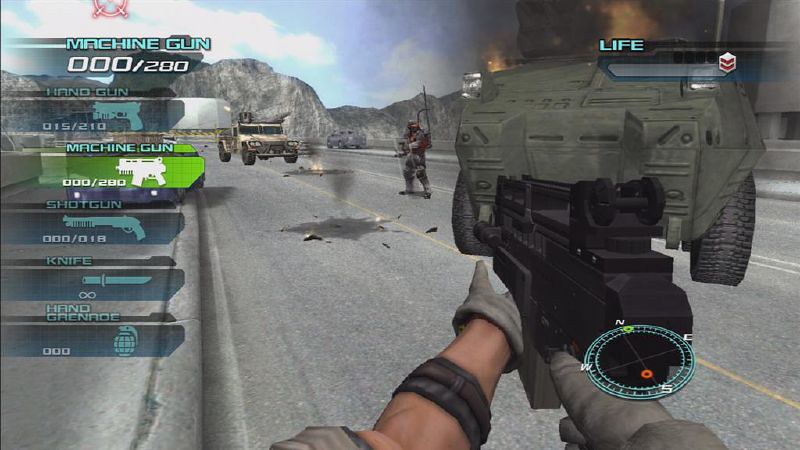The still image captures a moment from a first-person shooter video game, presenting the game from the perspective of the player. The player's arms, clad in tactical gear, are visible as they grip a large caliber, black firearm with both hands. The weapon appears menacing and powerful, ready for action. Above the weapon, a formidable armored vehicle with gray plating dominates the scene, indicating a likely focal point or objective within the game.

On the left side of the screen, a blue text display reads "Machine Gun," accompanied by an ammunition count of "00 out of 280," suggesting the player has depleted their current magazine which originally held 280 bullets. Below this, a weapon selection interface is visible, listing "Machine Gun," "Shotgun," "Knife," and "Hand Grenade," with the "Machine Gun" option highlighted in green, signifying it is the currently equipped weapon.

In the top right corner, a blue label reads "Life," next to which is a health meter and a shield gauge, indicating the player’s current vitality and defensive status. These elements provide crucial information about the player's in-game condition, enhancing the immersive experience of this virtual battlefield.